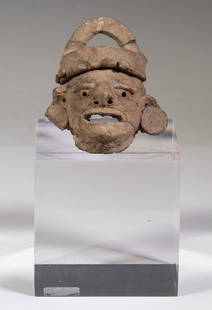The image depicts a detailed stone carving of an ancient artifact, possibly representing a man's head. The head is brown in color, reminiscent of dirt, with intricate details that give it a somewhat worn and weathered appearance. The artifact sits prominently on a translucent, frosted glass cube stand that adds a modern yet minimalistic display element, while slightly obscuring what's behind it.

The face of the statue is uniquely shaped, with prominent large eyes and a wide nose. The mouth is slightly agape, allowing a peek inside, which seems unintended for a solid statue, suggesting it might be an AI-generated image. The head is adorned with an arched, egg-shaped helmet that is thicker on the forehead. The ears are pressed close to the head, each earlobe adorned with large, ancient-style plugs or earrings, although part of the right earring appears broken.

Despite the seemingly authentic and historical aesthetic, the lighting and angles of the image look slightly off, reinforcing the impression that this could be an AI recreation of an ancient artifact. The entire scene is set against a gradient gray background, which provides a neutral backdrop that emphasizes the artifact's detailed features.